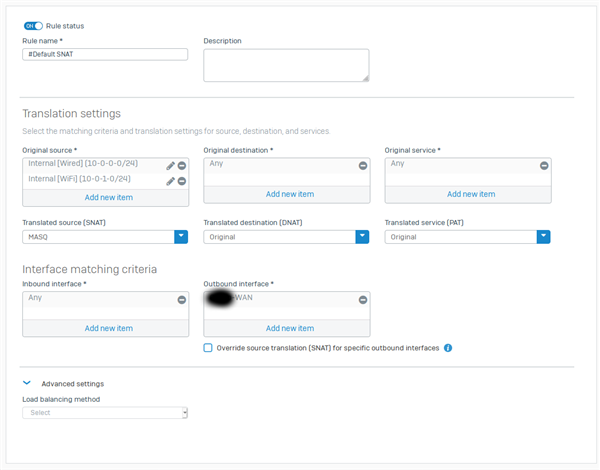This image features a screenshot from a user’s computer, displaying a configuration page for network rules. The page highlights the status of the rule, which is indicated as 'On.' The rule is identified by the name '#default SNAT.' 

In the section labeled 'Description,' there appears to be an editable text box. Moving down, the 'Translation Settings' area is presented, detailing various original and translated settings. These include 'Original Source,' 'Original Destination,' and 'Original Services,' followed by 'Translated Source (SNAT),' 'Translated Destination (DNAT),' and 'Translated Service (PAT).'

Further down the page, the 'Interface Matching Criteria' section shows fields for 'Inbound Interface' and 'Outbound Interface.' The 'Inbound Interface' field is set to 'Any,' while the 'Outbound Interface' field is obscured by a blurry black circle, likely for privacy purposes. 

Finally, at the bottom of the screenshot, there is the 'Advanced Settings' section, which mentions a 'Load Balancing Method' accompanied by a dropdown menu for selecting various options.